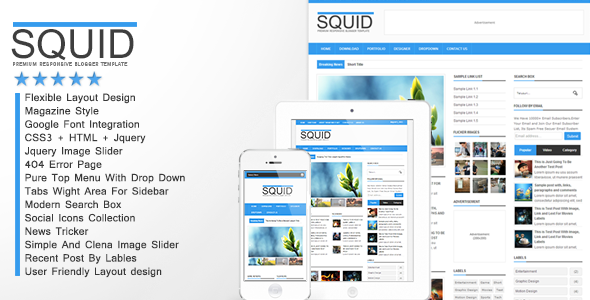The image features a webpage template with a minimalist, gray background. On the left side, a prominent blue horizontal bar spans about an inch and a half across the screen. Beneath this bar, bold black capital letters state "SQUID" followed by "Premier Responsive Blogger Template." Below the text, five blue stars are arranged in a horizontal line, indicating a rating. Further down, a vertical blue bar separates the left section from the right.

To the right of the vertical blue bar, there is a detailed black text list highlighting the features of the template:
- Flexible layout design
- Magazine-style format
- Google Font integration
- CSS3 and HTML compatibility
- jQuery and jQuery image slider
- 404 error page
- Pure-type menu with dropdown tabs
- A designated white area for the sidebar
- Modern search box
- Social icon collection
- New ticker
- Simple and clean image slider
- Recent post display by labels
- User-friendly layout design

On the right side of the image, there is a depiction of the template as it would appear on a web page, along with a screenshot of the template displayed on a mobile phone.